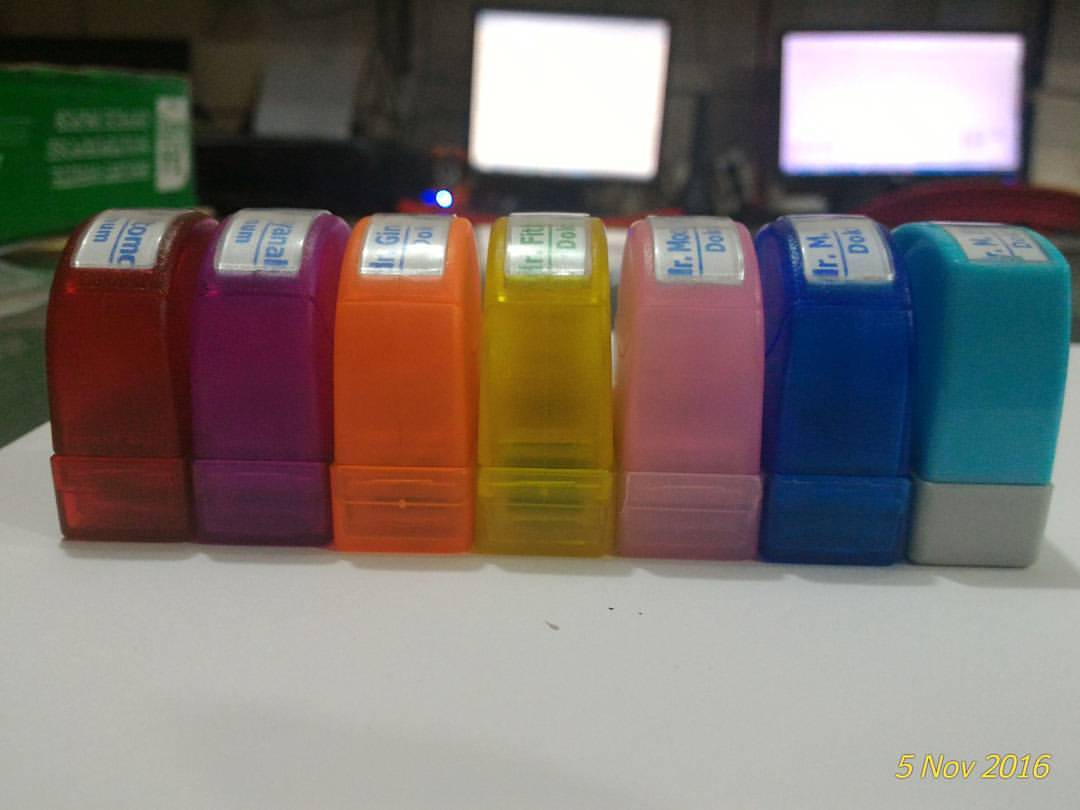In this indoor color photograph taken on a white countertop on November 5, 2016, there is a row of seven colorful dispensers, possibly tape dispensers or pill containers. The dispensers are neatly aligned from left to right, each featuring a consistent color with a gray sticker on top displaying blue writing, albeit illegible. The sequence starts with a red dispenser, followed by purple, orange, yellow, pink, royal blue, and Tiffany blue. Notably, the Tiffany blue dispenser has a gray bottom, unlike the others, which are uniform in color. Behind the dispensers, two bright white computer screens are visible on the right side with a dark green box featuring white writing on it in the upper left corner of the image. The date "5 NOV 2016" is overlaid in the lower right corner of the photograph.